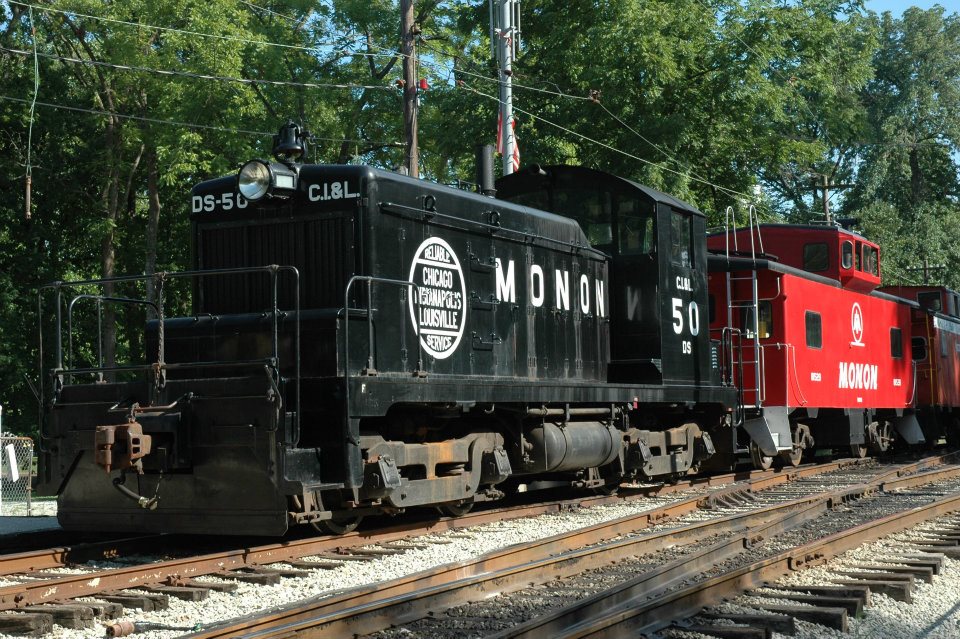The photograph captures a beautifully maintained section of old train tracks flanked by small white pebbles and lined with rusted brown rails. Dominating the image is a train with two distinct cars, the forefront featuring a black locomotive marked with "DS-50," "C.I. and L.," and a large circular emblem reading "Chicago, Indianapolis, and Louisville." This black engine has white letters and numbers, including "M-O-N-O-N" and "50," prominently displayed. Immediately behind it is a vibrant red car, adorned with a white bell symbol within a circle and marked again with "M-O-N-O-N." The tracks beneath the train are lined with white pebbles, complemented by darker pebbles filling the spaces between the metal rails. The backdrop comprises tall, overhanging trees with glimpses of blue sky peeking through the foliage. Electric and telephone lines stretch across the background, supported by a light grey metal pole and a wooden pole, adding to the historical ambiance of the scene. The meticulous detail of the train and its surroundings offers a nostalgic glimpse into a bygone era of railway travel.